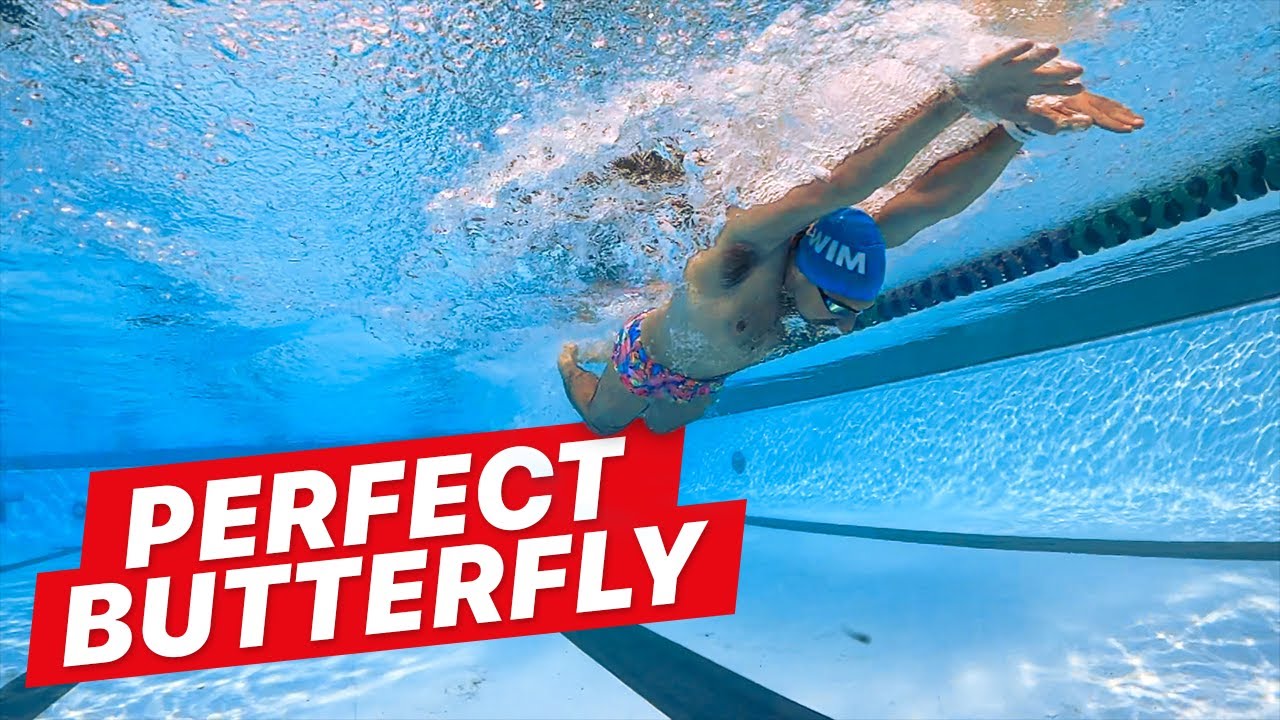This striking photograph captures a man swimming just below the surface of a pool, performing a perfect butterfly stroke. The swimmer is positioned centrally in the image, moving diagonally from the middle towards the top right. He appears to have just kicked off the pool edge, his arms stretched above his head and cupped together, creating an impressive splash as they break the water's surface. He is wearing a blue swim cap with white lettering that reads "swim", goggles, and multicolored floral-print swim trunks. The pool water surrounds him in cool shades of blue, with the black stripes of the pool lanes and a lane separator rope visible in the background. Bubbles rise above the swimmer, enhancing the dynamic movement captured in this underwater moment. In the bottom left corner of the image, the text "perfect butterfly" is prominently displayed in white lettering against a red background. The photograph not only highlights the swimmer's form and technique but also emphasizes the vibrant, colorful environment of the swimming pool.